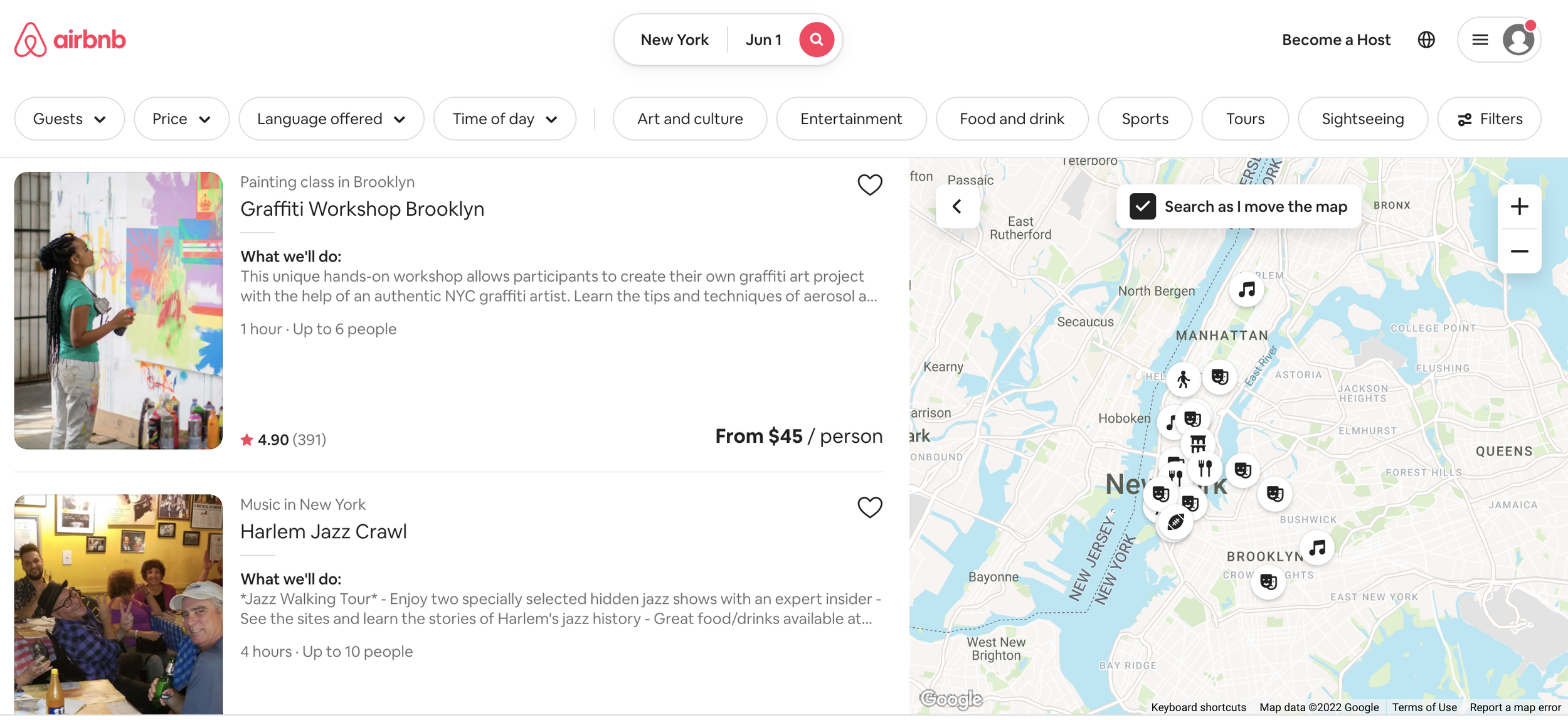This screenshot captures a search result page from the Airbnb website, focusing on experiences in New York for June 1st. On the left side of the page, two specific listings are displayed. The first listing is a graffiti workshop in Brooklyn, a painting class priced at $45 per person. This experience boasts an impressive rating of 4.9 out of 5 stars, based on 391 reviews. The second listing is the "Harlem Jazz Crawl," a walking tour centered around jazz music, accommodating up to 10 people over a duration of 4 hours, though the price is not visible in the screenshot.

On the right-hand side of the page, a map illustrates the locations of these experiences within New York City. The map features zoom controls (+ and -) in the upper right corner, allowing users to adjust the view for more detailed exploration of available activities.

At the top of the page, various filters are available to refine the search results, including options for guests, price, language offered, time of day, sport and culture, entertainment, food and drink, sports, sightseeing, tours, and more. Users can also log into their accounts or opt to become hosts via options provided in the top navigation bar.

Overall, this Airbnb webpage provides a user-friendly interface for discovering and booking unique experiences in New York City.